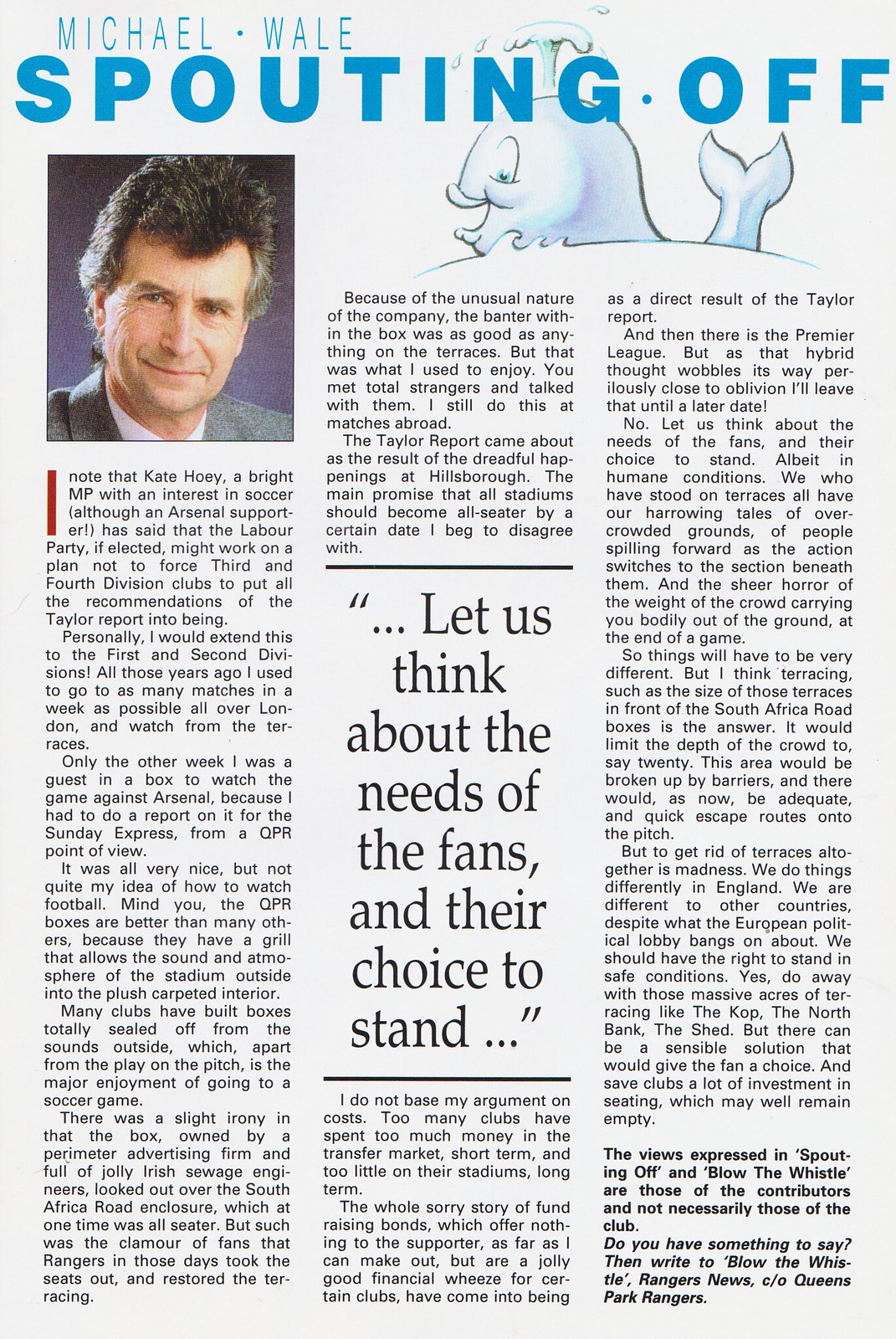The image is a vertically oriented clipping from an old newspaper or magazine featuring an article by Michael Whale. At the very top, in blue text, it reads "Michael Whale," followed by "Spouting Off" in bold, all-caps blue letters. To the right of these titles is a cartoon illustration of a smiling whale spouting water. Below the title on the left side, there is a small portrait of Michael Whale, a man in his 50s with short, spiky brown hair, wearing a gray suit and a white dress shirt, sporting a smiling, bemused expression. The article consists of three columns of dense text. A notable excerpt in the center, highlighted for emphasis, states, "Let us think about the needs of the fans and their choice to stand." The article discusses legislation potentially removing terraces from soccer stadiums, with Whale critiquing this move, articulating that doing away with terraces would be problematic. He references Katie Huey, an MP with an interest in soccer, who suggested that the Labour Party might not enforce all the recommendations of the Taylor Report for the 3rd and 4th Division Clubs. Whale extends this notion to the 1st and 2nd Divisions, sharing his personal experiences and opinions on the matter.